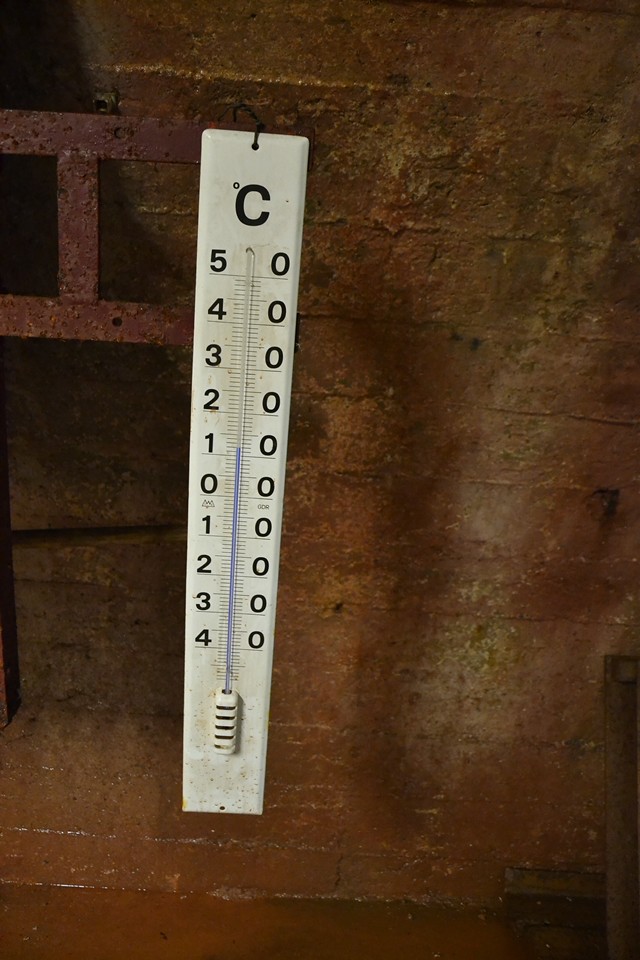The photograph features an antique Celsius thermometer affixed to an aged, plastered-over brick wall. The thermometer, with a range from minus 40 to positive 50 degrees Celsius, contains blue liquid that serves as the mercury. Enclosed in a wrought iron frame, the thermometer stands out starkly against the weathered background. 

The thermometer itself is a dirty white, showing signs of age with mildew stains visible up to the minus ten degree mark. The temperature scale is marked in black numbers on a white background, with the left side presenting increments of 5 down to 0 and negative 10 going up to minus 40. The right side of the scale shows increments from 50 to 0. The brick wall behind it appears quite old, with some moisture seeping onto the floor beneath it. The presence of the wrought iron frame, which is a flattened cast iron piece, adds a rustic charm to the scene.